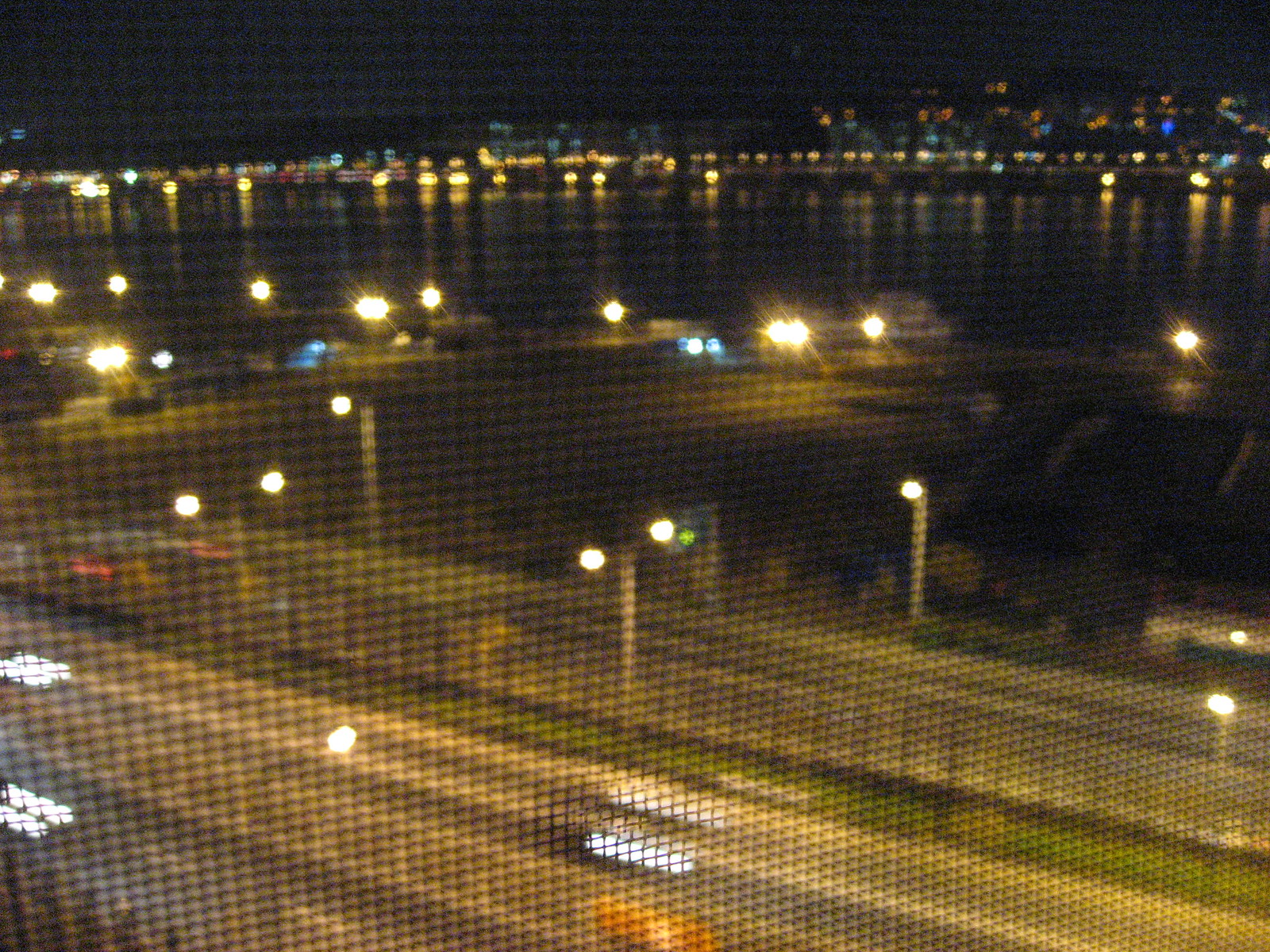This night-time photograph captures a sprawling urban landscape from an elevated vantage point, approximately a hundred feet above the scene. The dark sky serves as a backdrop to a vibrant cityscape adorned with a myriad of colorful lights—blues, oranges, and yellows. Dominating the foreground, a major highway divided by a grassy median runs across the image, with traffic visible in both directions. Streetlights dot the roadway, interspersed with light poles, casting an ambient glow.

A distinctive feature is the body of water, likely a harbor or a wide river, situated behind one of the highways. The water's surface mirrors the city's bright lights, adding another layer of luminescence to the scene. Docks and possibly boats are discernible along the shoreline, contributing to the industrial ambiance. There’s mention of potential loading scaffolding along the opposite shore, though high-rise buildings could also explain the towering silhouettes.

The photograph is taken through a black metal grill, visible as a slightly blurred crosshatch pattern, which adds an element of depth and frames the bustling nocturnal landscape below. The city lights in the background form a distant, shimmering horizon against the inky night sky.